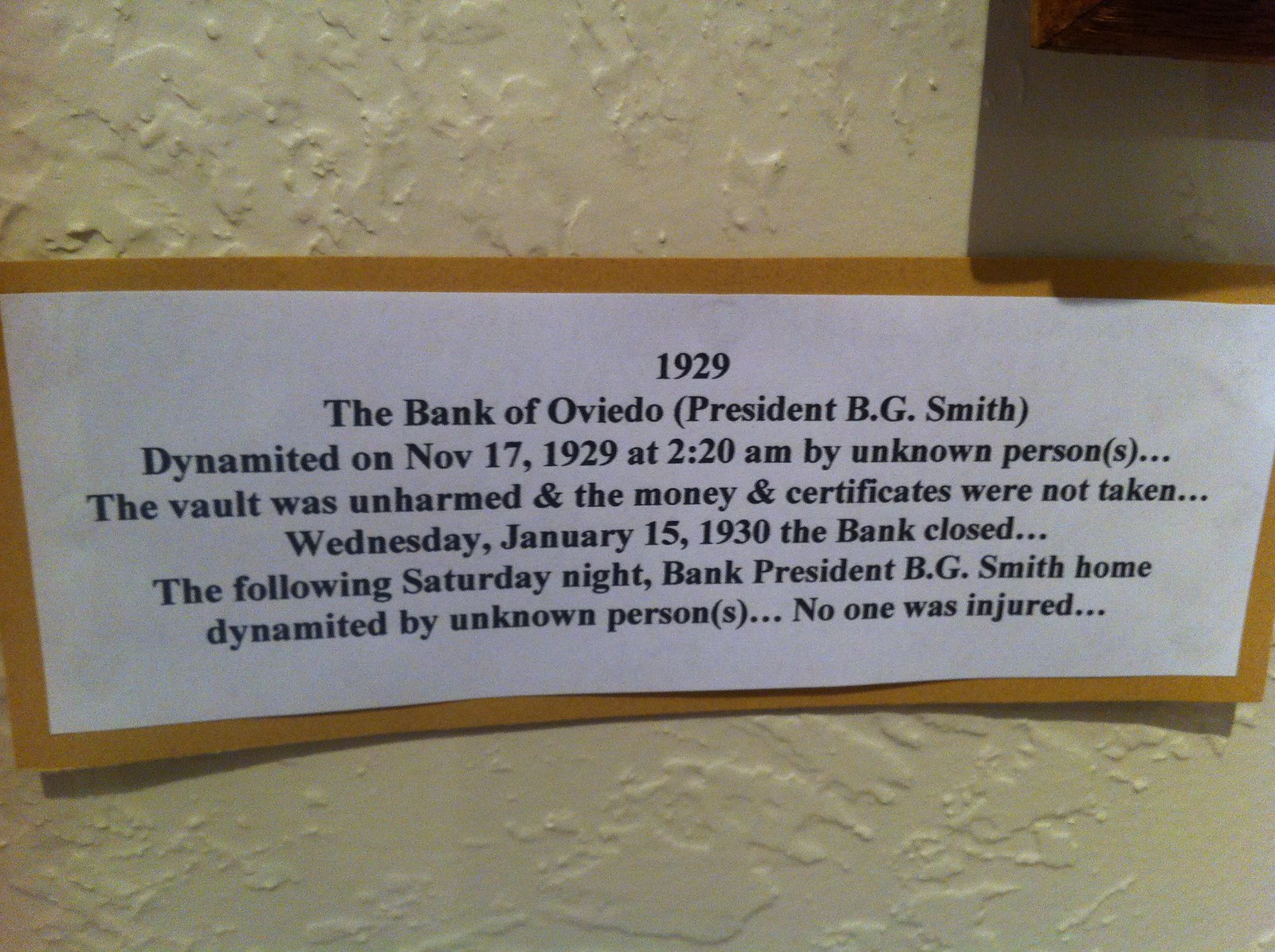The image depicts a piece of white paper framed by brown paper, hanging against a beige stucco wall. The paper contains plain black text with the following details: “1929, The Bank of Oviedo (President B.G. Smith), dynamited on November 17, 1929, at 2:20 a.m. by unknown persons. The vault was unharmed and the money and certificates were not taken. Wednesday, January 15, 1930, the bank closed. The following Saturday night, Bank President B.G. Smith’s home dynamited by unknown persons. No one was injured. For more information, visit www.fema.gov.” A shadow is visible in the top right corner of the image, but its source is unclear.